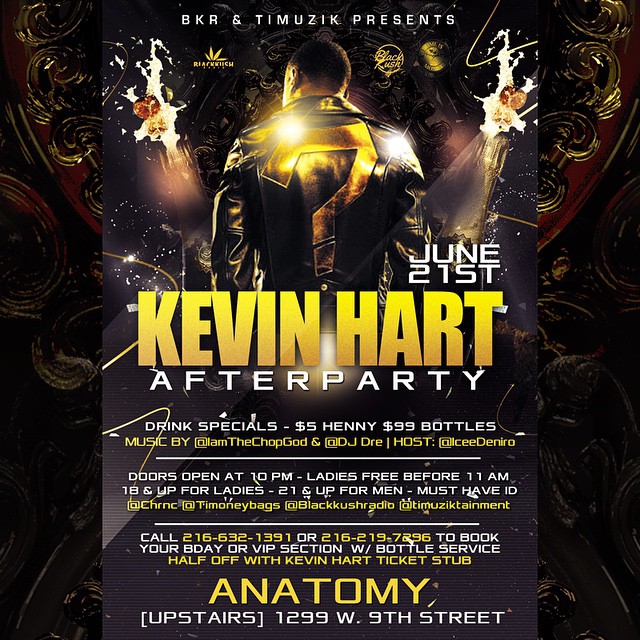The image is a rectangular advertisement with a slightly taller-than-wide orientation, featuring a dark background of black, maroon, and gold tones. At the top center, in prominent white font, it states "BKRNT Music Presents," although "Music" is misspelled as "MUZIK" in another instance. Just below, the text announces "June 21st" in the upper right corner. The center showcases the upper torso of a man with brown skin, facing away from the camera. He sports a short haircut and is clad in a black leather jacket adorned with a golden question mark on the back. 

Centered below this image, "Kevin Hart" is boldly printed in gold, followed by the words "After Party" in white. Beneath that, the text lists drink specials including "$5 Henny" and "$99 Bottles." The event features music by "@IAM The Chop God" and "@DJ Dre," and is hosted by "Ice E.E. De Niro."

Additional details include "Doors Open at 10 PM," "Ladies Free before 11 AM," with entry requirements stating "18 and up for ladies," "21 and up for men," and "Must Have ID." At the bottom, contact information is provided for booking birthday or VIP sections with half-off bottle service using a Kevin Hart ticket stub. The venue "Anatomy upstairs" is located at "1299 West 9th Street."